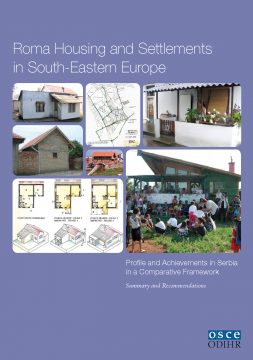This image is the cover page of a pamphlet titled "Roma Housing and Settlements in Southeastern Europe." The background is purple and features two lines of text. The cover showcases various images related to Roma housing: the top left displays a mobile home, while the bottom left quadrant highlights a detailed diagram of a house, identifying spaces like the living room and bedroom. A central map possibly depicts Southeastern Europe, and the center-right image captures a festival gathering. Additionally, on the top right, there's a picture of a white house with flowers on the balcony and an awning. The bottom of the cover further mentions "Profile and Achievement in Serbia in a Comparative Framework," indicating a focus on both the specifics of Roma settlements and broader regional comparisons. This guidebook provides detailed information about Roma residential setups and community life in Southeastern Europe.